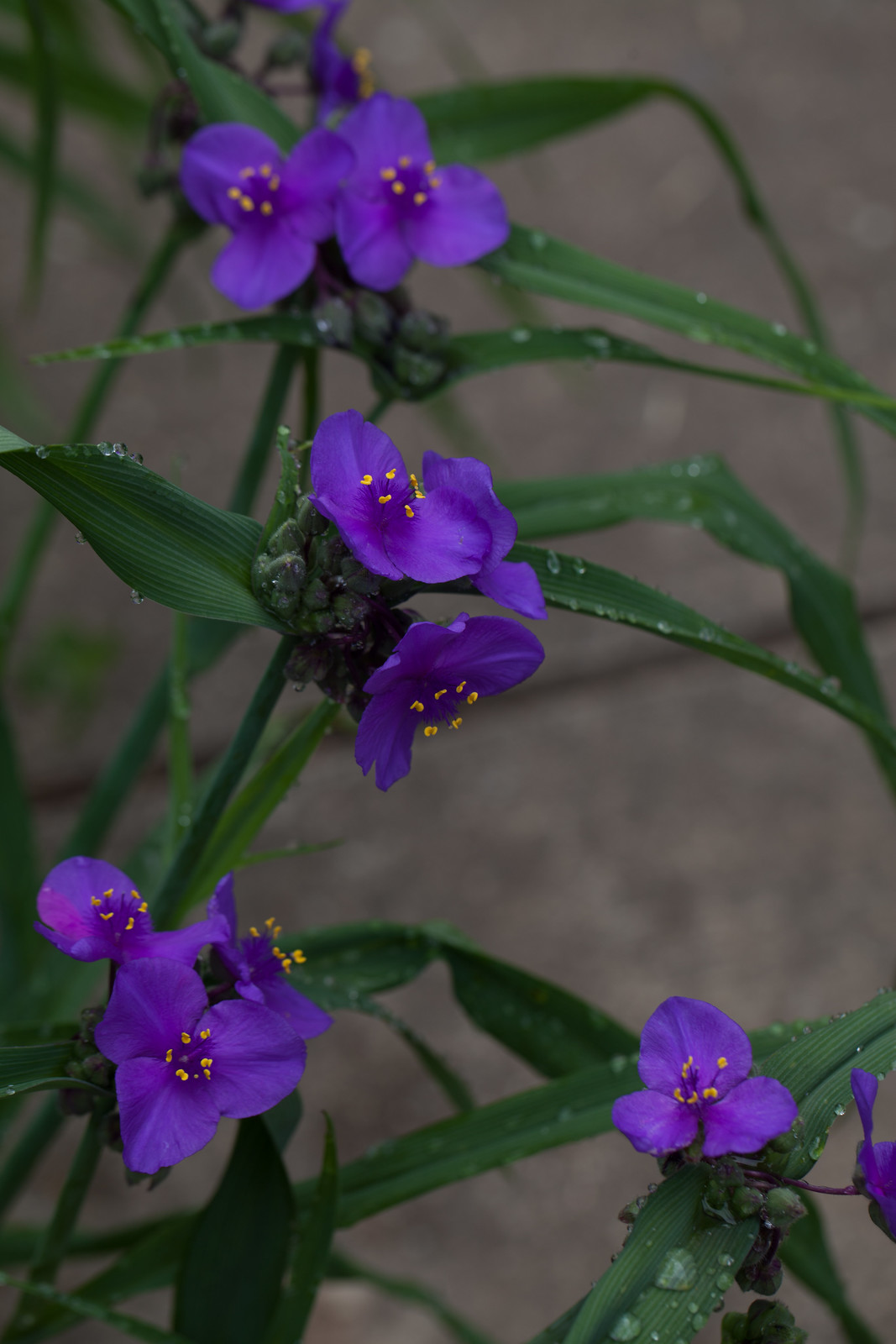This close-up photograph captures the intricate details of a flowering plant with vibrant purple blooms, each featuring three petals and bright yellow pollen buds in the center. The flowers, some of which are still budding, are adorned with tiny white droplets of dew on their flat, triangular green leaves, adding a fresh, morning-time atmosphere. The scene is set against a gray, rocky background, possibly stone or concrete, with variations in lighter shades that highlight the flowers' vivid colors. The flowers are visible in clusters at the top, center, and bottom of the image, showcasing a rich tapestry of natural beauty in a small, intimate space. The detailed, zoomed-in view allows one to appreciate the fiber bands running across the leaves, enhancing the textural depth of the photograph.